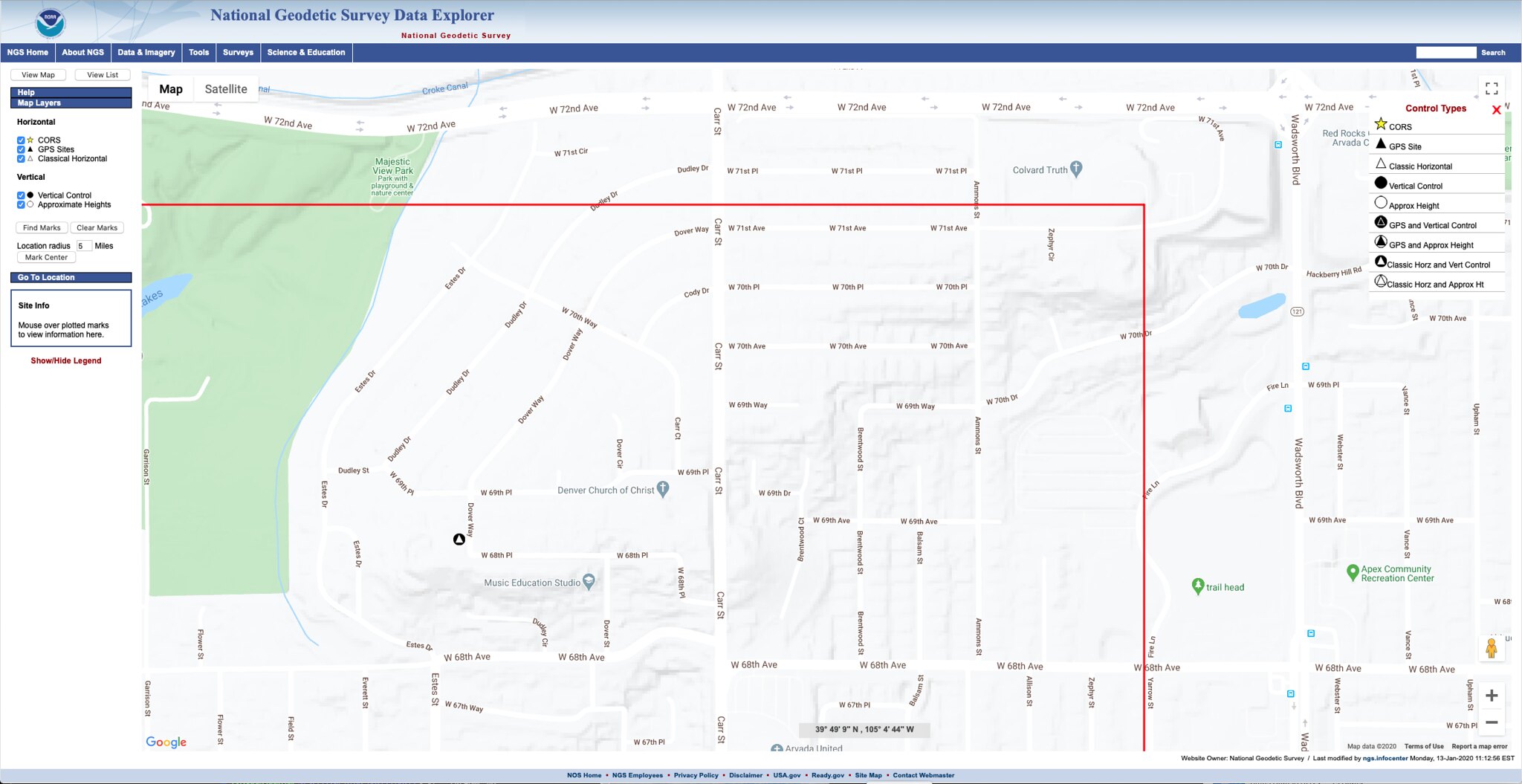The image depicts a detailed street map with extensive small printed text, making it difficult to read specific details. At the top, the text "National Survey Data Explorer" is visible, suggesting that the map is derived from a national survey. The map has a white background with numerous black lines and letters scattered throughout at various angles, representing different streets or data points. 

A green box on the map likely indicates a park or a designated green space. Additionally, a red line runs diagonally, forming part of a square, possibly highlighting a specific area or route of interest. On the left side of the map, there's a scale bar for distance measurement, and on the right side, there are other markings and labels, though they are tiny and difficult to discern.

The map is bordered by a navy blue color at the top and a light blue color at the bottom, adding a frame-like effect to the overall appearance. This image combines the elements of a street map with data visualization, likely providing insight into the results of a national survey.